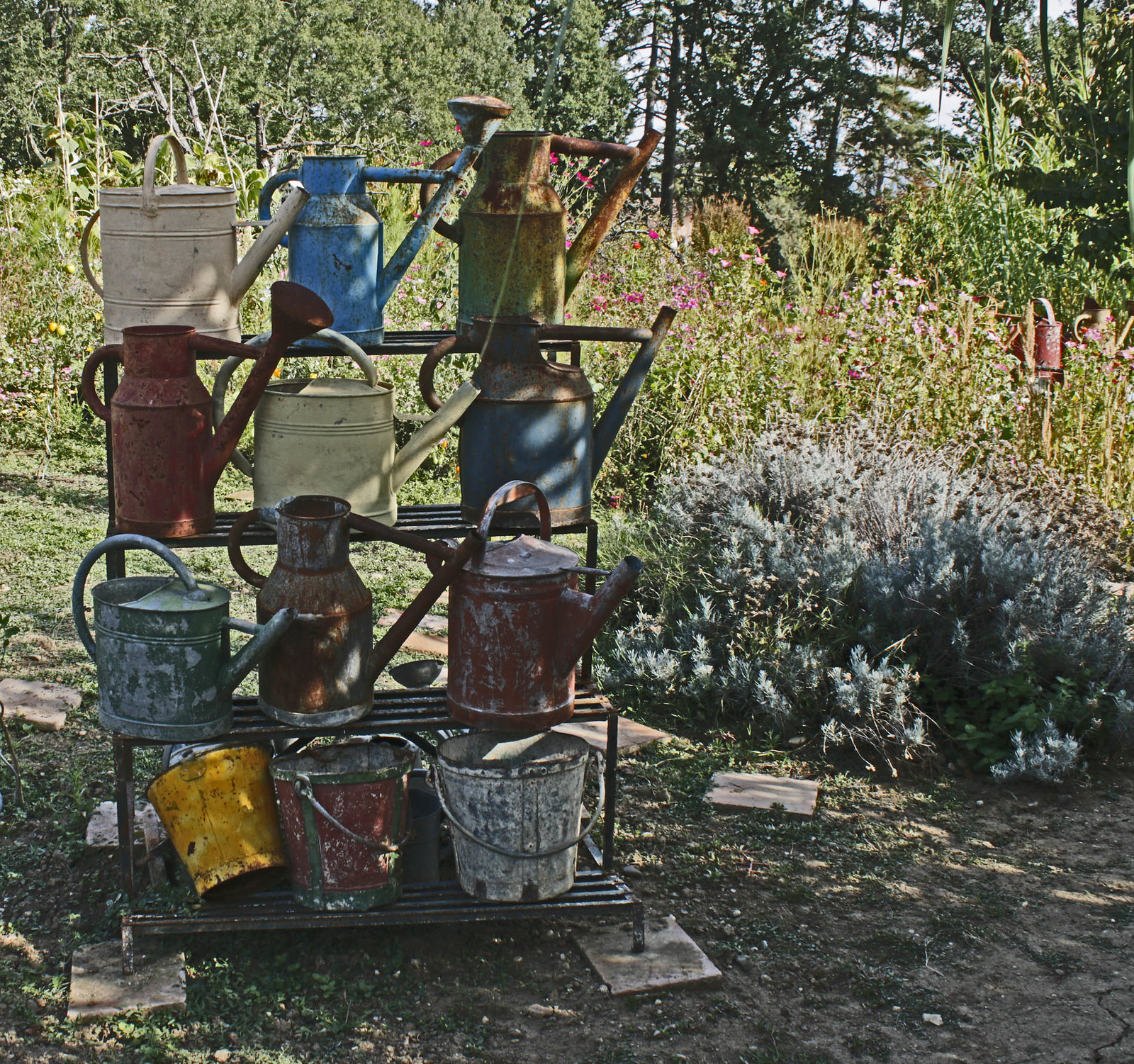This detailed outdoor color photograph features a weathered metal shelving unit occupying the left half of the image, loaded with various garden items. The sturdy frame, made from narrow beams, holds four layers of rusted and worn watering cans and jugs, all facing rightward. On the bottom shelf, three pails are arranged: yellow on the left, red in the center, and gray or white on the right.

Moving up, the second shelf displays three watering cans: light gray on the left, brown in the middle, and red and white on the right. The third shelf holds another collection: an off-white can on the left, a blue can in the middle, and a green and brown rusted can on the right. The top shelf mirrors this diversity with a white can on the left, a light blue can in the middle, and a half green, half brown can on the right.

The items on the shelving unit, which is black, feature a mix of colors including beige, blue, green, red, silver, and yellow. All appear significantly weathered, with rust and dark markings indicating their age and exposure.

Beneath the unit lies a faded patch of green grass flanked by brown earth. Surrounding the frame on the ground are five small square objects, with what appears to be a spike protruding through at least two of them. To the right, a lush green bush is present, accompanied by tall pink flowers and various green foliage.

In the background, taller trees and a small expanse of grey sky peek through the upper right hand corner. Sunlight bathes the flowers and trees in illumination, contrasting with the shadow-clad foreground, suggesting the photo might have been taken around sunrise or sunset on a pleasant day.